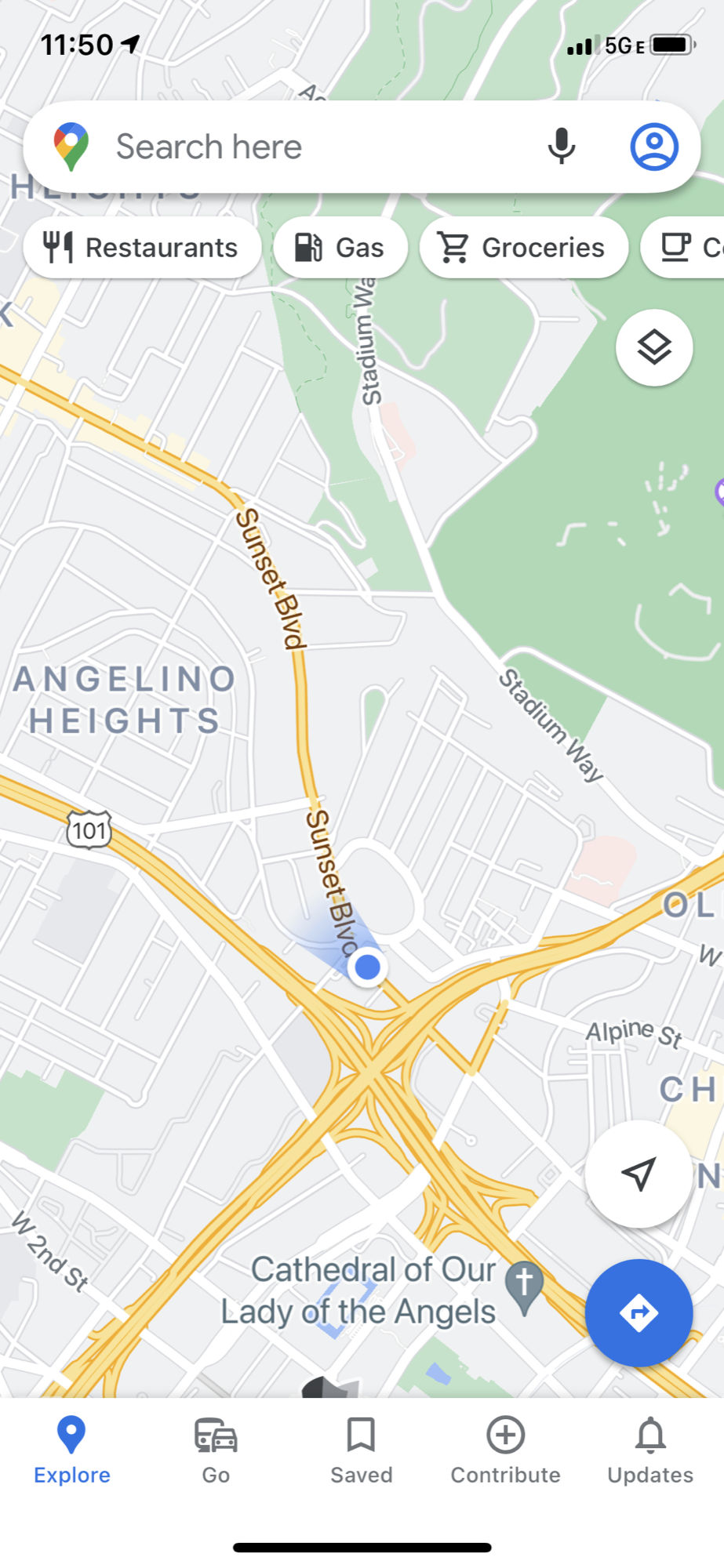A Google Maps screenshot taken at 11:50 AM displays a semi-charged battery at approximately 75% and a signal strength of three out of four bars on 5G. The interface includes a "Search here" prompt along with quick access icons for restaurants, gas stations, and groceries. The map highlights the vicinity of Sunset Boulevard, Angelo Heights, Stadium Way, Cathedral of Our Lady of the Angels, and Alpine Street. Below the map, tabs for "Explore," "Go," "Save," "Contribute," and "Updates" are visible, along with a prominent black bottom bar. A blue circle with a directional arrow and a white circle with a directional arrow are also featured. The central area of the map showcases a network of streets converging with prominent on-ramps and off-ramps marked in yellow, while the surrounding areas depict gray streets interspersed with green grassy zones.